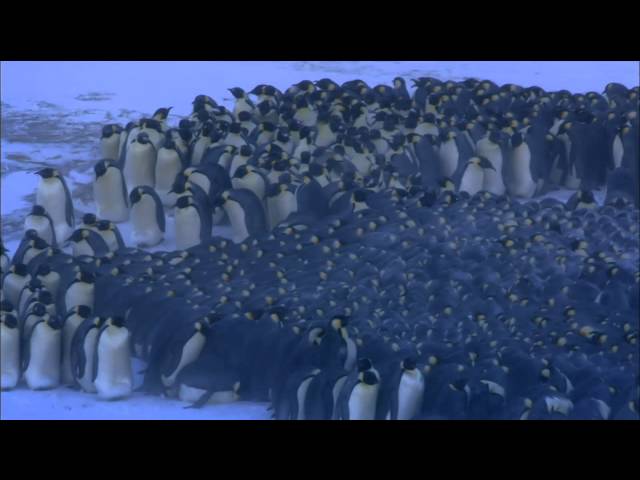A large group of emperor penguins, predominantly black on their backs and white on their chests, are densely huddled together on a snowy, frost-covered ground. Their black heads, adorned with distinctive yellow patches on the sides, peek through the tight formation at the top of the image, creating a pattern of black and yellow dots. Towards the left, the penguins are more spread out, revealing individual behaviors such as heads tilting up or down and some penguins facing forward, exposing their white chests. There is a noticeable black strip across both the top and bottom edges of the photo. In the middle bottom section, it's difficult to discern whether the area shows tightly packed penguins or water, as it appears as a solid blue space with yellow dots resembling their faces. The overall scene suggests the penguins are huddled together to keep warm in the dimly-lit, cold environment.